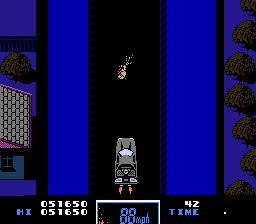A small, square image captured from a computer or phone screen displays a digital racing game. The bottom 10% of the image features a black strip populated with various numeric data. Above this strip, the game itself unfolds against a royal blue background, dominated by a thick black road running vertically up the center of the screen.

Situated at the bottom center of this road is a sleek sports car, viewed from above, primarily gray in color with visible fiery exhausts streaking out from its rear. A piece of scattered debris lies further up the road, directly in the vehicle's path. On either side of the road, the royal blue background continues, interspersed with narrower vertical black strips.

To the left of the main road, a yellow-brick building is visible from an aerial perspective, appearing distinctly separate from the game’s roadway. On the right side of the road is a patch of dark green shrubbery.

The bottom strip of the image contains digital readouts, with the numbers "051650" repeated twice, one above the other, on the left side. To the right, a white "42" is displayed above the word "TIME" in blue. Centrally located within this strip is a white rectangle displaying the vehicle's speed as "88 MPH" in a highly digital font.